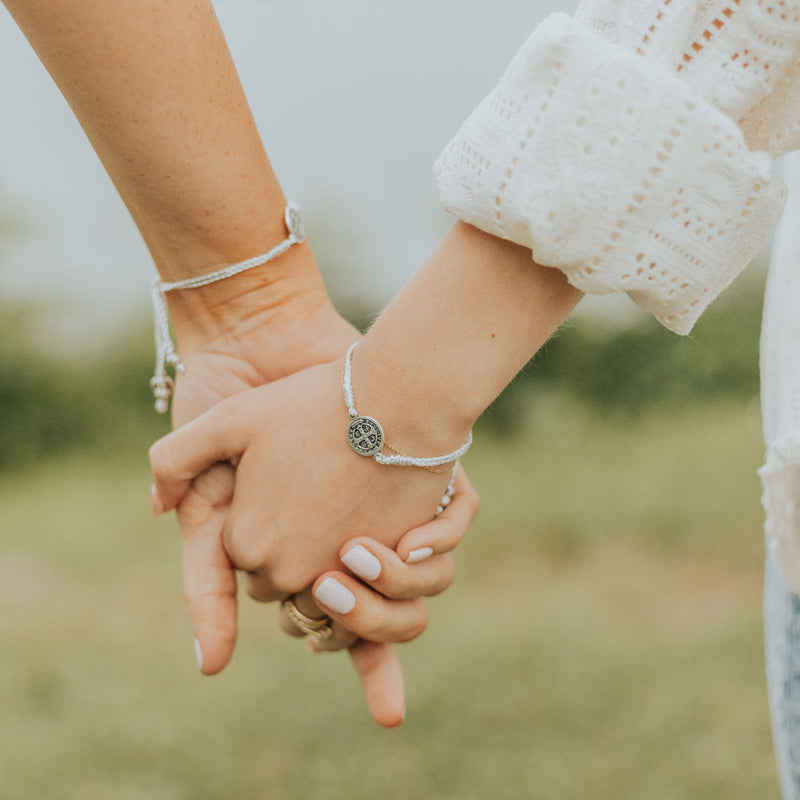This detailed photograph, likely taken by a wedding photographer, captures an intimate moment of a couple holding hands against a blurred background of a green and brown pasture with a treeline. The focus is on their interspersed fingers, revealing their matching thin macrame bracelets adorned with silver charms—a Celtic cross and white beading—that elegantly dangle from their wrists. The woman's hand, featuring short-cropped nails painted in a simplistic white polish, also showcases a gold wedding ring with a diamond. Her outfit is partially visible, with a rolled-up sleeve of a white cuffed shirt adorned with a lacy eyelet design. The man's hand, slightly larger, complements the scene with his matching bracelet and more neutral nail polish. The closely framed image zeroes in on the delicate details of their connection, highlighting the emotion and subtle elegance of the moment.